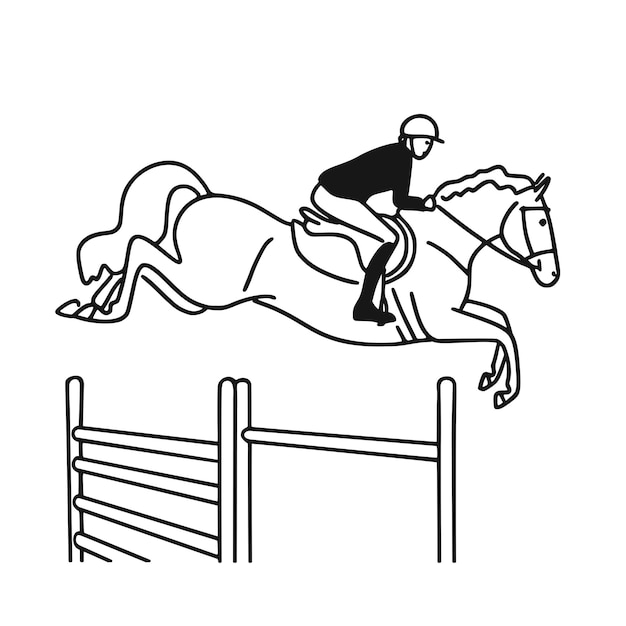This black and white illustration depicts a show jumper on a horse mid-leap over a complex obstacle. The background is completely white, emphasizing the stark black outlines of the subjects. The horse, with both legs extended in the air, appears to be jumping over a set of two adjacent obstacles. On the left, there is an H-shaped structure with four parallel bars, while on the right, there is a similar H-shaped structure with a single, higher bar. The jockey, clad in a long-sleeved black shirt, white pants, black knee-high boots, and a white helmet, grips the saddle and reins tightly, guiding the horse over the barriers. The dynamic positioning of both horse and rider suggests a moment of intense concentration and skill, making the scene vividly dramatic despite its monochromatic simplicity.